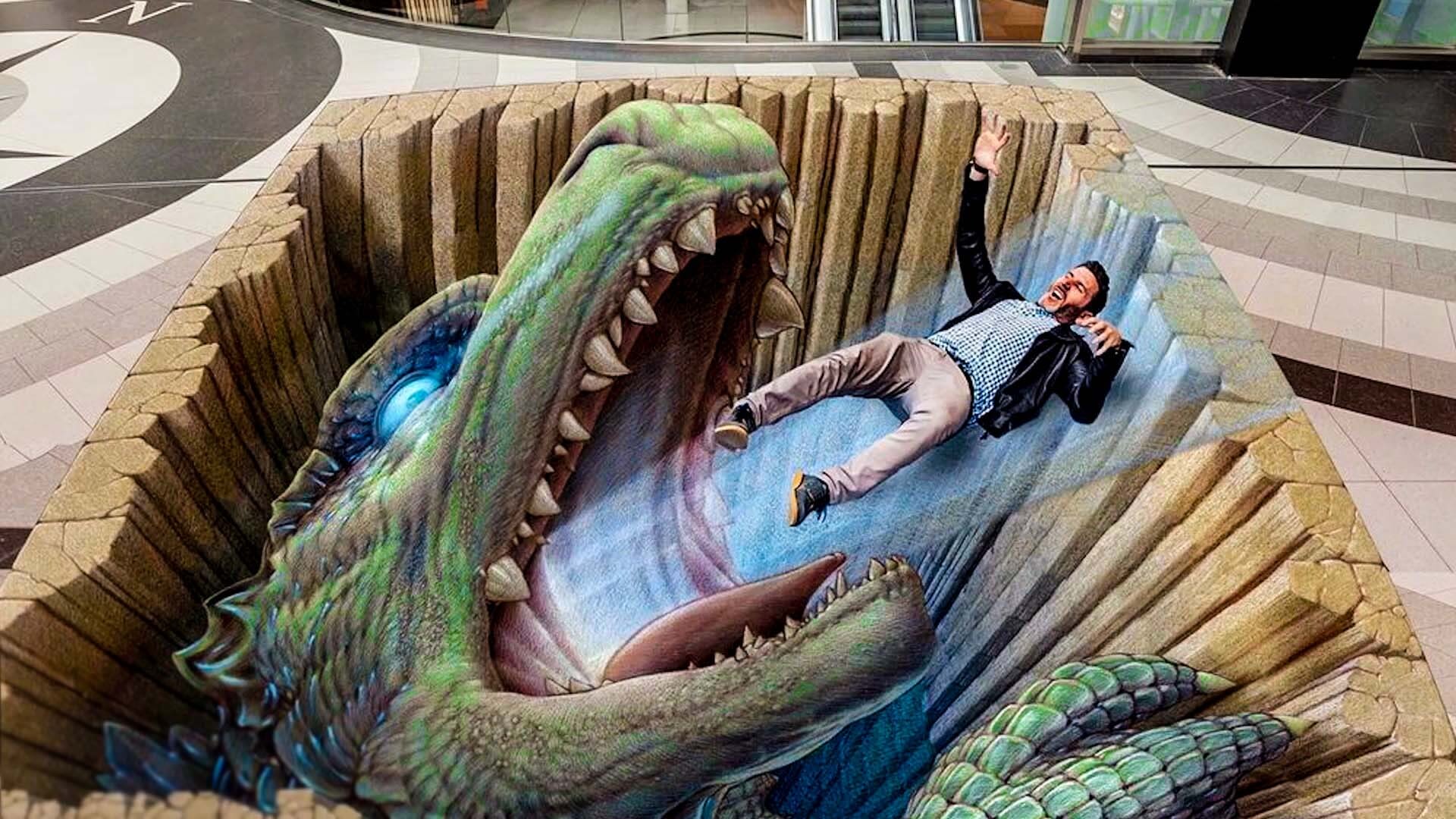The image is an intricate, computer-generated optical illusion artwork painted on the floor of a public space such as a shopping center courtyard. The primary focus of the scene is a remarkably detailed and somewhat realistic depiction of a green dragon, characterized by opalescent, scaly skin, jagged teeth, and a luminous blue eye. Emerging from a wood-enclosed pit strewn with various colored concrete slabs forming a circular mosaic pattern, the dragon's mouth is agape, emitting a ray of blue light. This light ensnares a man, dressed in khaki trousers, black shoes, a blue and white plaid shirt beneath a black leather jacket, giving the illusion that he is being drawn into the dragon's gaping mouth. The man appears to have a horrified expression as he lies on his back with arms raised. Additionally, part of the dragon's claw can be seen grasping at the wooden planks surrounding the pit. The overall composition gives the surreal yet highly detailed impression of a dragon consuming a person, complemented by tiles on the floor that range from cream to dark brown, enhancing the depth and realism of this fantasy illustration.